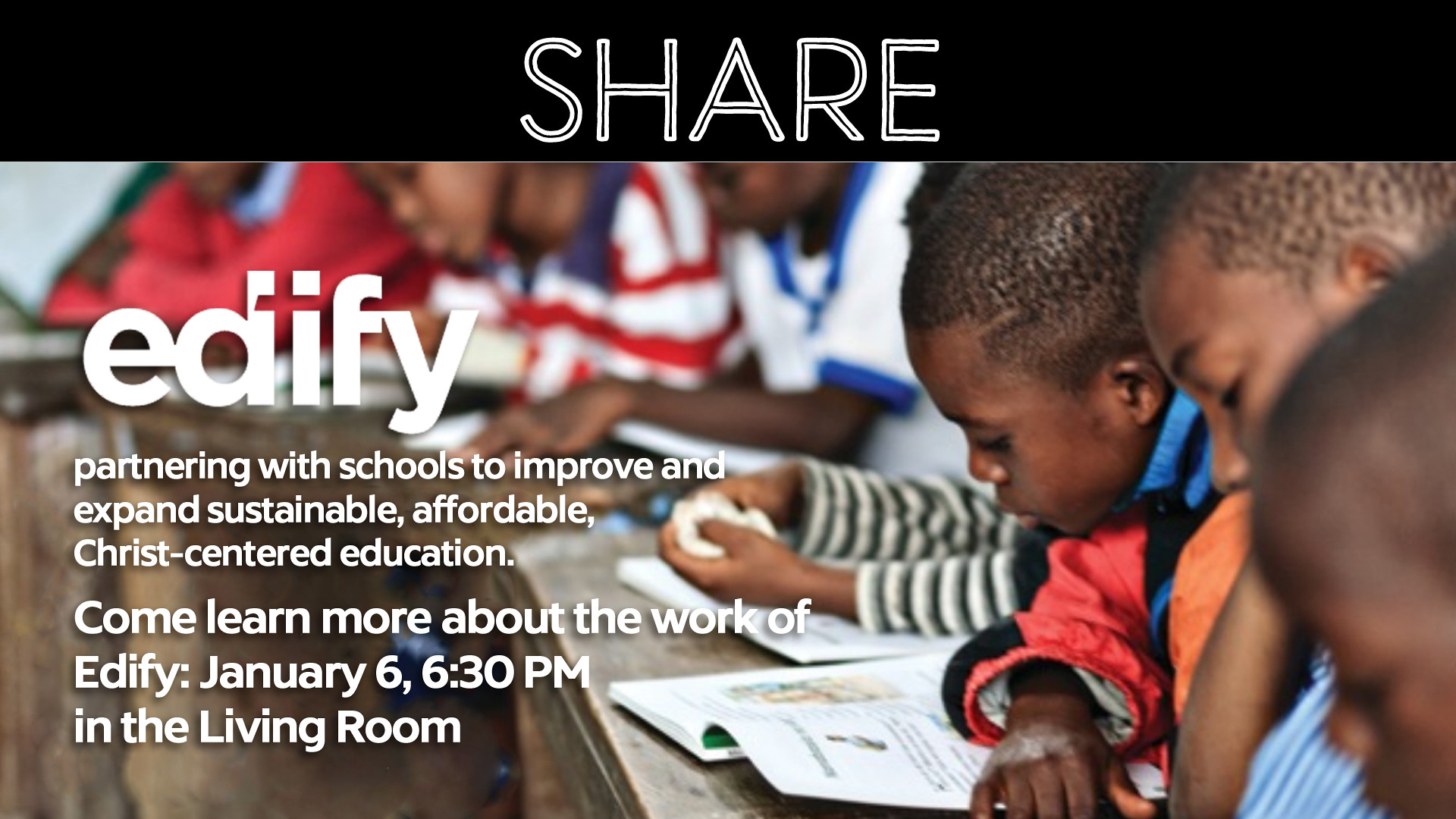The image is a wide, high-definition photograph primarily showcasing a group of young African-American boys diligently studying in a classroom. They are seated in a row at desks, with open books in front of them, their gazes intently focused on reading. Most of the boys are dressed in coats and long sleeves, suggesting a cooler environment. 

The top fifth of the image features a prominent black bar with the word "SHARE" in bold white letters. Superimposed on the left side of the photo is another message, which reads: "EDIFY. Partnering with schools to improve and expand sustainable, affordable, Christ-centered education. Come learn more about the work of EDIFY, January 6th, 6:30 p.m. in the living room." This appears to be an invitation to an informational event about the organization's mission and work.